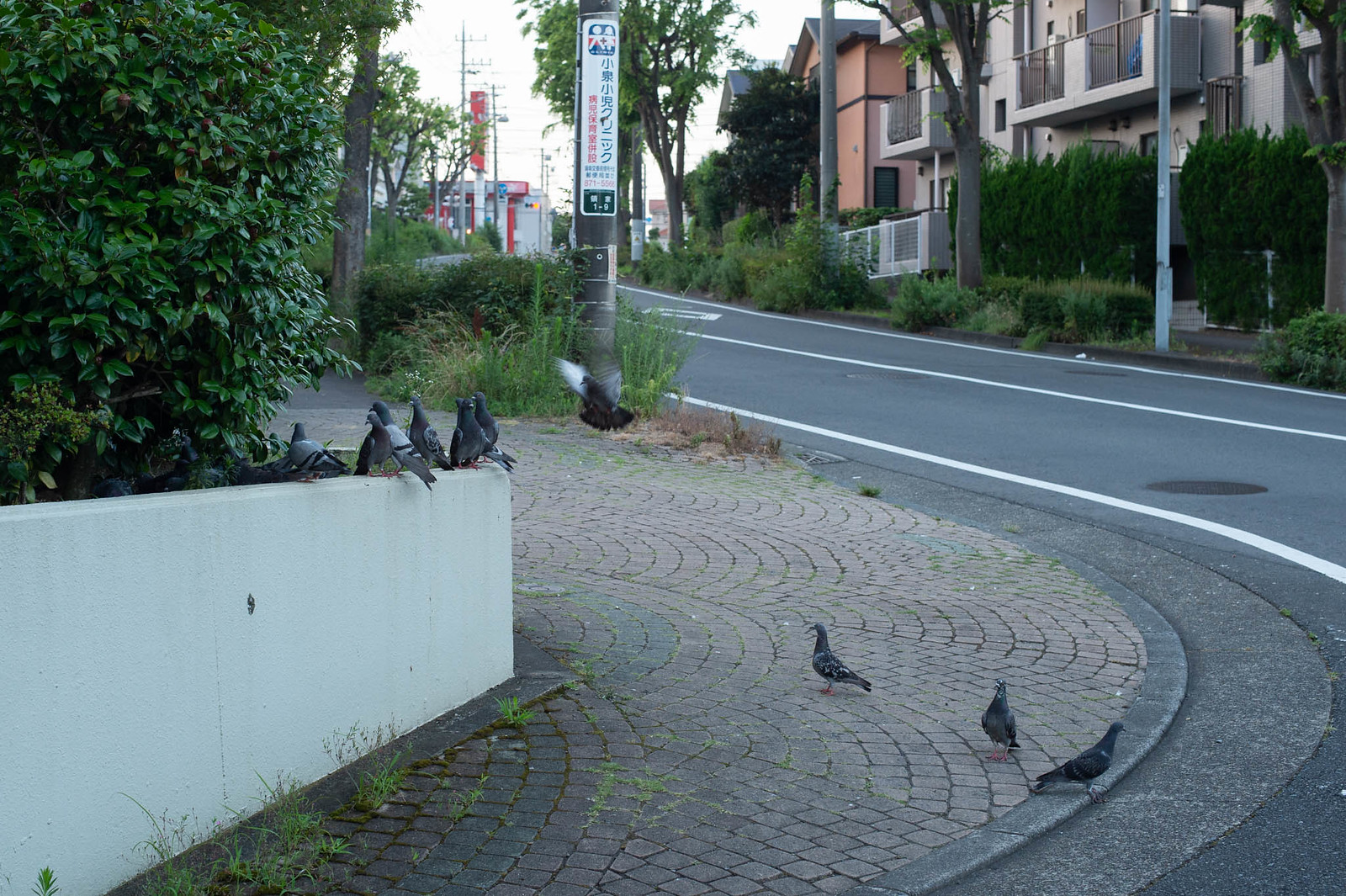The daytime photo captures a quaint small-town street scene on a curved road. On the left side of the road, a brick sidewalk with faded pink pavers leads into an area bordered by lush green bushes and a short white wall. Grey pigeons populate this area, with several perched on the wall, some on the sidewalk, and one walking into the street. One pigeon is also seen flying towards the wall. The road features three white stripes, including one in the middle. On the right side of the road, amidst more green brush, stand a few tall, two-story apartment buildings, one white and another red. Further down the street, a gas station with a white sign topped by a red emblem and a covered port with pillars can be seen in the distance. The sky is bright and white, providing a clear backdrop for the scene. There are also several grey and white street signs, and trees with brown trunks and light green leaves are in front of the houses, adding to the picturesque setting.